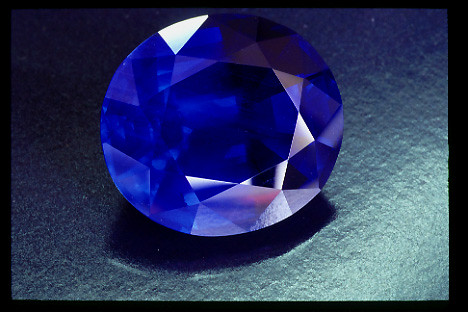The image shows a vivid, faceted gemstone that's a deep, dark blue color, situated on a rough-finished, coated tabletop or counter. The surface beneath the gem transitions from a dark gray to almost black at the top, becoming lighter towards the bottom, which might be an effect of the lighting. This substantial gemstone, cut into numerous reflective facets, captures and refracts light, resulting in vibrant white reflections on its diamond and triangular sections while some facets appear almost black. The most striking and vivid blue part of the gem is on the left side, with more variations in color appearing on the right and bottom, suggesting that the light source is positioned off-frame to the bottom right. The gemstone, resembling the shape and form of a traditional ring stone but without a setting, rests centrally and prominently in the image, with a black border framing the scene.